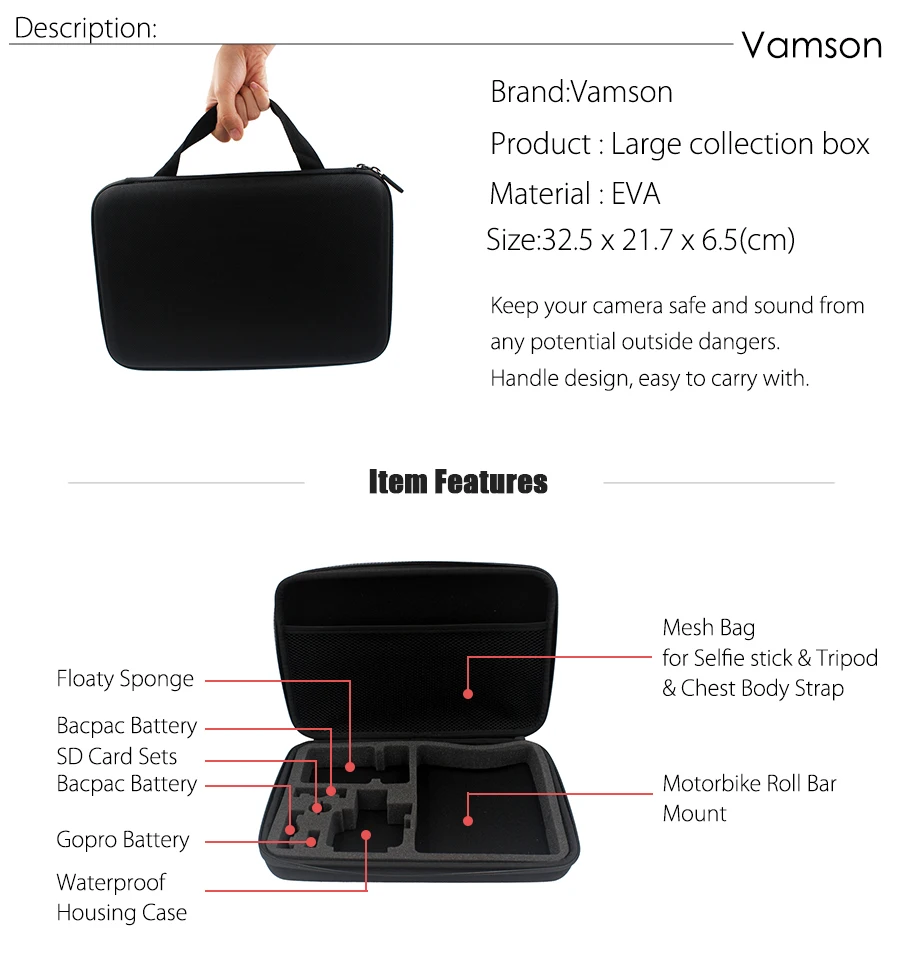Screenshot of a VAMSIN Camera Bag Product Description on a White Background

The screenshot showcases a detailed product description of a VAMSIN brand large collection bag, designed specifically for carrying camera equipment. The bag is made from durable EVA material and measures 32.5 x 21.7 x 6.5 centimeters. 

In the upper left corner of the image, bold black lettering on a white background highlights the VAMSIN brand name and the product description. A human hand is shown holding up the carrying bag, indicating its size and ease of use. The bag's design focuses on keeping your camera safe and secure from potential hazards, with a robust handle for easy carrying.

Key features are listed below in bold lettering under “Item Features”:
- The case can be opened to reveal a floaty sponge, providing additional protection.
- There are specific compartments for various accessories including a backpack battery, SD card sets, GoPro battery, waterproof housing case, motorbike roll bar mount, and a mesh bag suitable for a selfie stick and tripod.
- The case also includes a chest body strap for added convenience.

This detailed list comprehensively illustrates how the VAMSIN camera bag keeps your gear organized and secure.